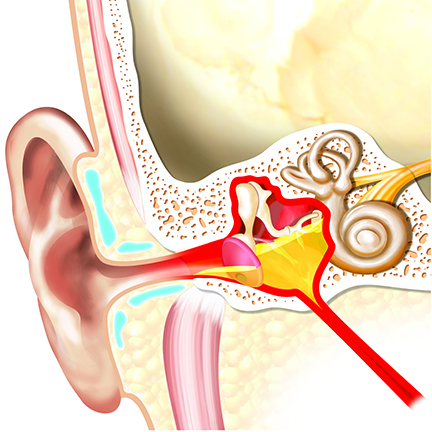This highly detailed illustration of the inner workings of the human ear, akin to something you might find in a medical textbook, showcases a variety of anatomical structures in vivid colors. The exterior of the ear is depicted in a tan or skin color, leading into the ear canal that transitions through shades of pink, red, and yellow. At the entrance of the canal, the coloration starts as skin-toned before becoming more intensely red a couple of inches in, signifying the deeper internal areas.

Within the ear canal, a red circular flap can be observed, possibly indicative of a vein or another structure. Surrounding it is a yellow substance that resembles earwax. Prominently featured is a snail-shaped, spiral structure in a tannish-brown color, representing the cochlea, the essential organ for hearing. Adjacent to the cochlea is a white and yellow porous, bone-like material, and above this is a yellowish-cream colored area.

Distinct pink tubes extend in various directions – one downward and another upward, potentially indicating the eustachian tube or other auditory pathways. The entire diagram is rich in color, utilizing hues of pink, white, beige, red, yellow, and even a hint of light blue immediately inside the ear canal. The background features spongy, porous material, likely depicting the surrounding cartilage or supporting structures of the inner ear. Overall, the illustration provides an in-depth, close-up view, capturing the complexity and intricacy of the ear's internal anatomy.